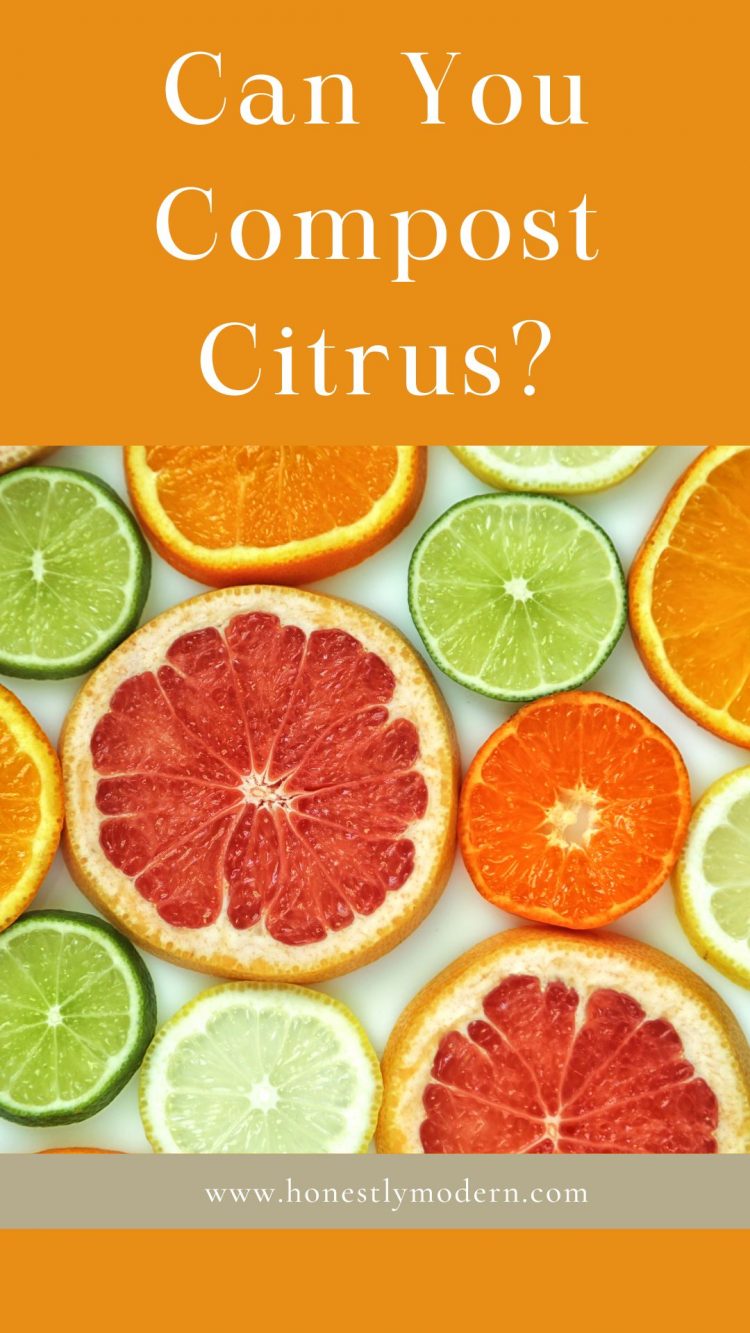The image, seemingly from an instructional website, prominently features the question "Can you compost citrus?" displayed in white text against a burnt orange background. Below the header, there's a visually striking photograph showcasing an assortment of different sliced citrus fruits arranged on a white plate. The selection includes vibrant orange oranges, dark pink grapefruits, tangy lemons, zesty limes, and potentially blood oranges or mandarins. Each fruit is meticulously cut into thin, flat slices and closely arranged together, creating a colorful mosaic. At the bottom of the image, against a thin grey strip, is the website URL: www.honestlymodern.com. The image combines informative elements with bright, contrasting colors, and the overall design suggests it aims to educate rather than serve as a comical piece.